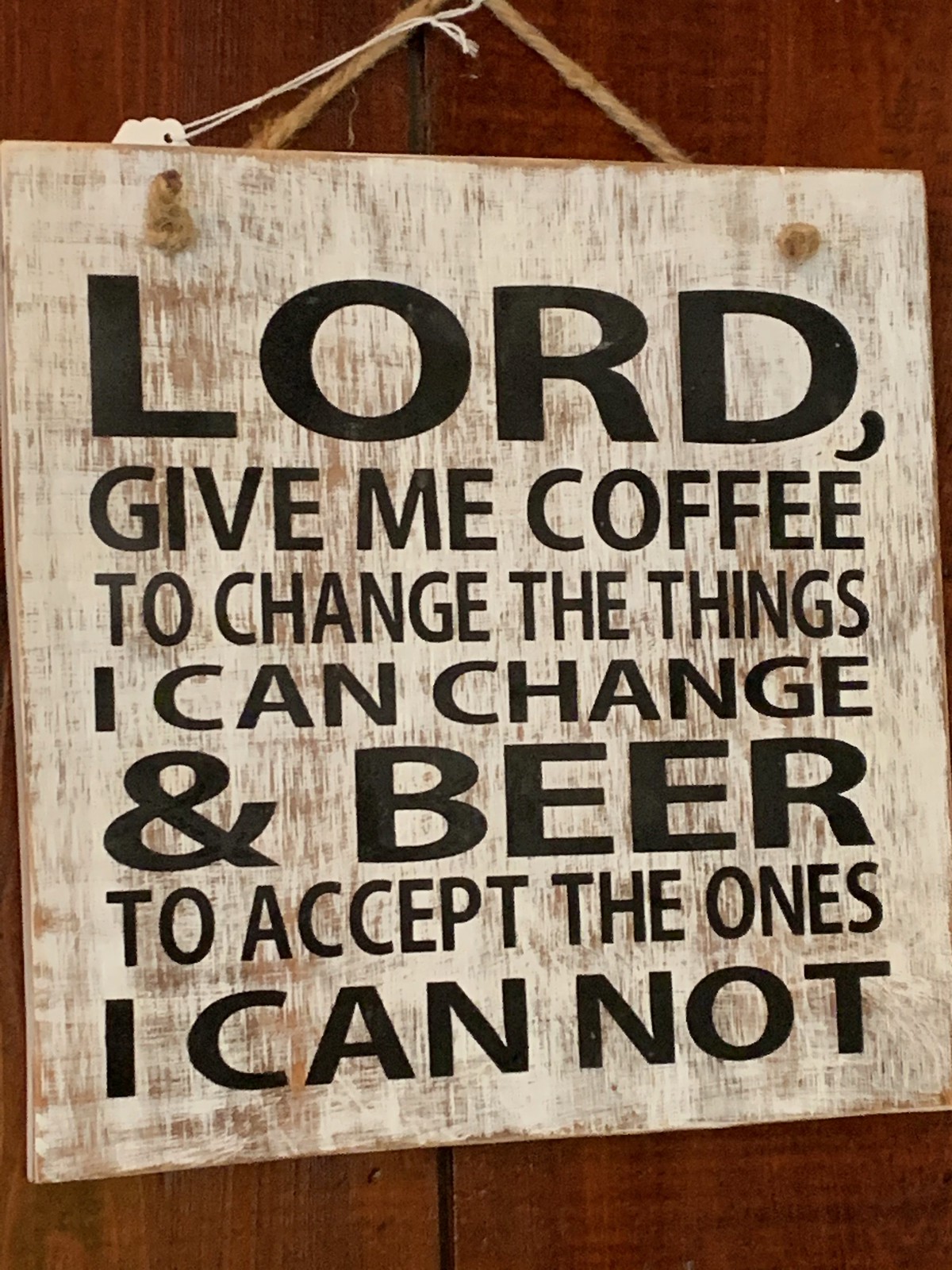A wooden plaque is securely attached to a rustic wooden wall, featuring a humorous yet reflective inscription. The sign reads, "Lord, give me coffee to change the things I can change and beer to accept the things I cannot." The message, written in large, clear black font, is easy to read and evokes a lighthearted approach to coping with life's challenges. This tidy, well-crafted plaque is designed to be a charming and visually pleasing addition to any space, offering a touch of humor and wisdom.